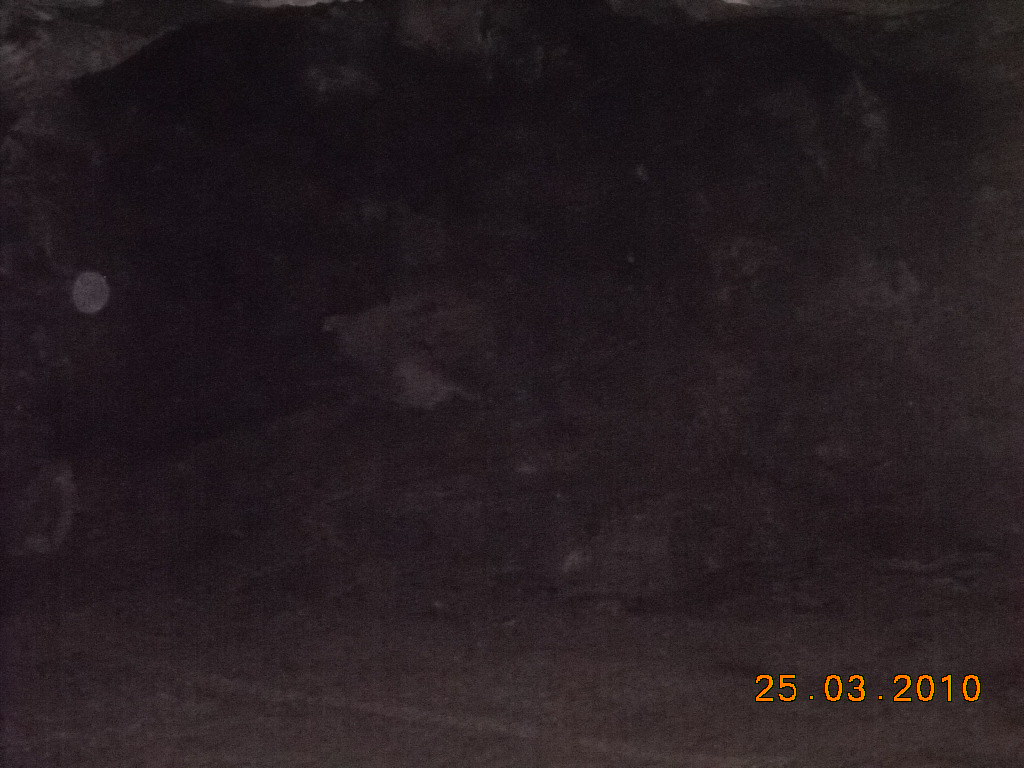A grainy, dark image with a timestamp of "25.03.2010" in the bottom right corner. The top left corner shows a bright white area, contrasting with smaller white splotches scattered in the center. To the left, a noticeable dot on the lens suggests the image is slightly dirty. The background appears gray and undefined, with the image marred by various splotches and marks, adding to its unclear, grainy appearance.